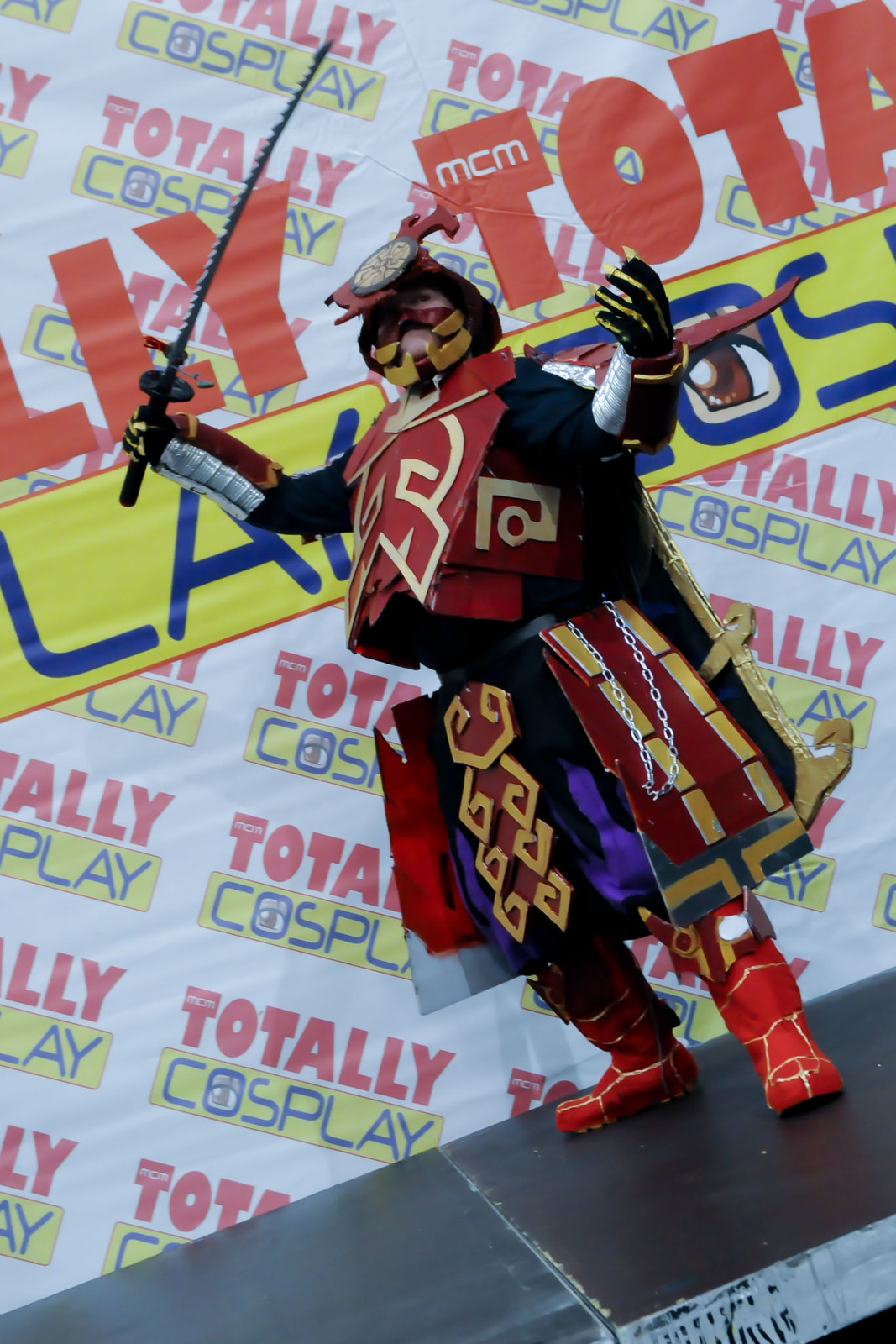At a London event called Totally Cosplay, a participant is depicted in an intricate and vibrant costume resembling a stylized Japanese samurai with manga influences. The character's identity is ambiguous, as their face is obscured by an elaborate red and yellow mask adorned with gold points extending towards the mouth. A striking headpiece featuring a round, black-edged design with gold trimming crowns their short black hair. 

The person's attire includes a prominent red and gold breastplate, complemented by black sleeves with silver cuffs and black and gold gloves. Their lower half is clad in black pants overlaid with a stiff, cardboard-like skirt comprised of red and gold panels, each with sharp golden points and decorative gold rectangles. A white chain drapes from the waist area, adding to the ornate aesthetic.

The ensemble is completed with red boots trimmed with gold. In the character’s right hand, they wield a black katana-like sword with white markings along the blade, enhancing the warrior appearance. The backdrop of the black stage features a banner proclaiming "Totally Cosplay," solidifying the event’s theme and setting.